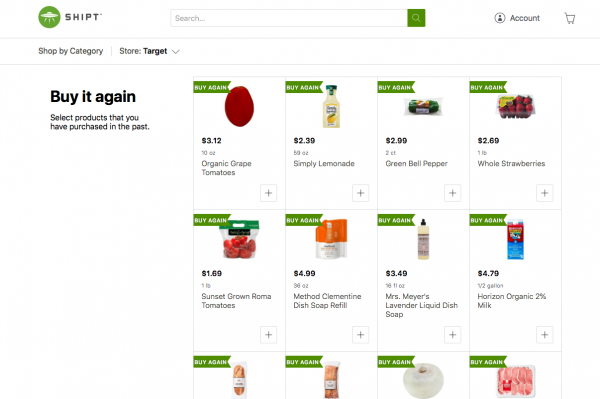The image is a screenshot of the Shipt app interface, showcasing a selection of available items from a Target store. In the upper left corner of the screenshot, the Shipt logo, a green circle with a white flying saucer icon, is prominently displayed next to a search bar. Just beneath this area, there are options labeled "Shop by category," "Store: Target," and "Buy it again." 

On the upper right side of the interface, there is an "Account" option accompanied by a shopping cart icon, which indicates that no items have been added yet. 

The main portion of the screenshot displays 12 rectangular product images arranged in a grid of four rows and three columns. Each rectangle contains a different item alongside its description and price. For example, in the upper left rectangle, there is an image of organic grape tomatoes priced at $3.12 for a 10-ounce container. Adjacent to this, the next rectangle features a bottle of Simply Lemonade, priced at $2.39 for a 59-ounce bottle. The Simply Lemonade is shown in its signature clear plastic bottle with a yellow liquid inside.

The remaining rectangles similarly showcase a variety of items available for purchase, though none appear to have been selected, as evidenced by the empty shopping cart icon in the upper right corner.